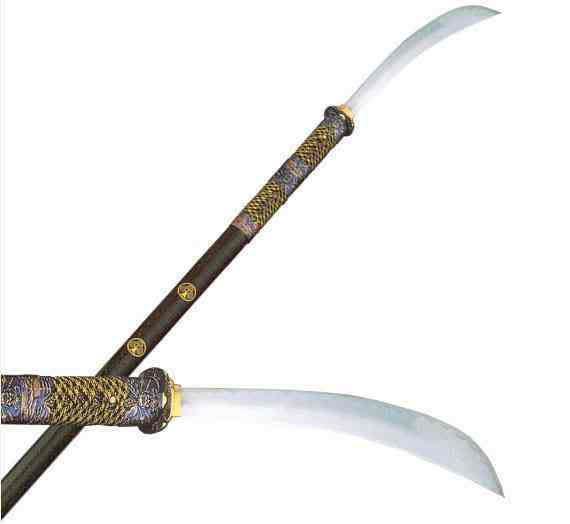This image features two intricately designed, medieval-style blade weapons displayed on a completely white background. The weapons share a distinct, almost identical design, highlighted by long, slender handles wrapped with gold embellishments and ornate features. One handle, appearing wooden and predominantly brown, showcases two small round gold emblems and some blue patterning with additional gold highlights. 

In the foreground, a close-up view reveals a detailed shot of the blade which is silver and pointed, curving gracefully into a sharp edge. The gold mounting at the junction where the handle meets the blade adds to the intricate design. In the background, you can see more of the second weapon, which is displayed diagonally from the lower left corner to the upper right corner. The blade of the background weapon appears longer and runs almost horizontally across the image.

Both weapons exhibit elaborations that suggest an ancient or medieval aesthetic. While the blade in the foreground showcases more detailed close-up features, including the top part of the handle with the gold wrap, the weapon in the background reveals the full extent of its handle and its characteristic embellishments, including the dual gold circles. The silver blades gleam against the white background, emphasizing their sharp, curved edges and intricate craftsmanship.